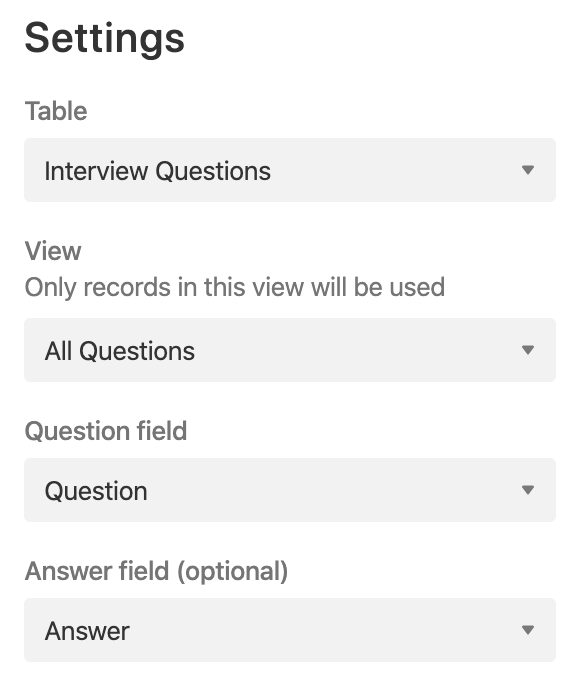The image appears to be a smartphone screenshot, potentially capturing a pop-up settings window. The background is entirely white with no borders. At the top, "Settings" is prominently displayed in bold, black letters. Below it, "Table" is written in large, gray letters, followed by a long horizontal gray bar. On this bar, "Interview Questions" is written in black on the left, accompanied by a downward gray arrow on the right.

The next section has a white background with gray text that reads "View." Beneath it, a description in gray letters states, "Only records in this view will be used." Below this, a bolded black text appears against a gray background, stating "All Questions," with a downward arrow to the right.

Further down, another white section features gray text that reads "Question Field." Underneath is a gray bar with black text, "Question," and a downward arrow on the right. The subsequent white section contains gray text, "Answer Field (optional)." The final gray bar at the bottom displays "Answer" in bold black text, with another downward arrow on the right. Throughout the image, text on white sections appears in gray, while text on gray sections is bolded in black.